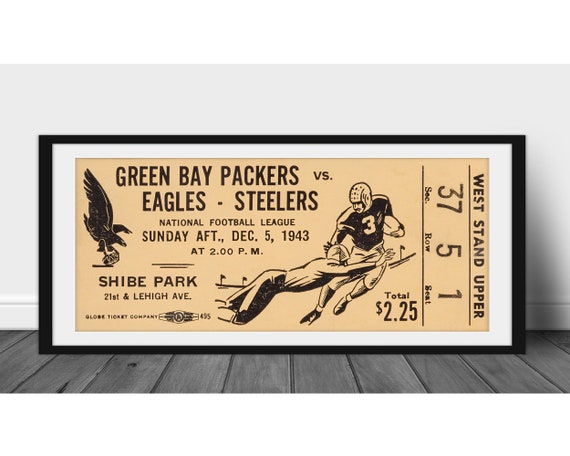The image depicts a large, framed, and poster-sized reproduction of a vintage game ticket, intricately detailed. The frame is black with white matting, highlighting the rectangular, tan-colored ticket which prominently displays the text "Green Bay Packers versus Eagles Steelers" in bold black capital letters. Below this, the ticket states "National Football League," followed by "Sunday Afternoon, December 5th, 1943," and the game time listed as "2 o'clock p.m." The ticket notes the location as "Sheeb Park, 21st and Lay Avenue," and features an advertisement for the "Glove Turkey Company" near the bottom. To the left, an illustration captures an eagle emblem, while to the right, two football players in vintage gear are shown: one evading a tackle with the ball in hand, adding dynamic action to the design. The ticket price, prominently visible, is stated as "$2.25," with additional details indicating "Section 37 Row 5 Seat 1, West Stand Upper."